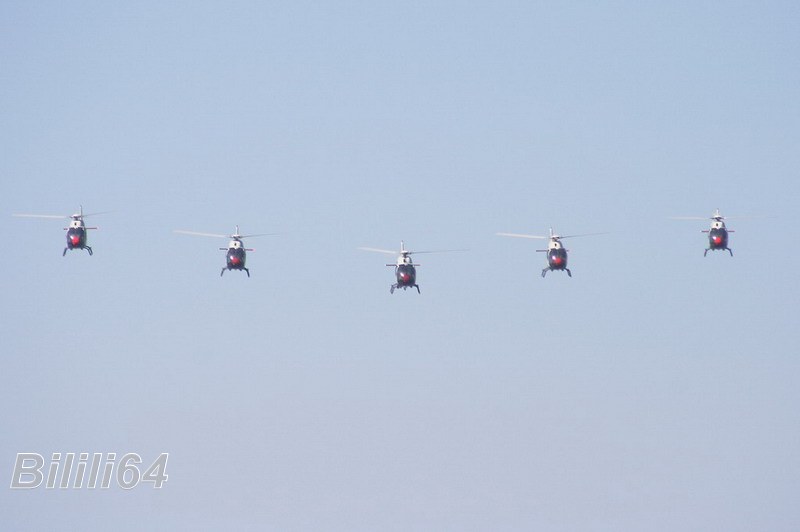The photograph captures a striking scene of five helicopters flying in a precise formation against a gradient blue sky that darkens slightly towards the top. Taken from another aircraft, the image shows the helicopters aligned in a shallow V or echelon formation, with the center helicopter slightly lower and the others gradually higher outwards. Each helicopter is characterized by a dark body with a black nose and a distinct red circle at the tip. The upper parts and propellers of the helicopters are white, and the motion of the blades is blurred, indicating their operation. There are no other visible elements—no clouds, structures, or terrain—just the expansive sky. In the lower left corner of the image is a watermark with sans-serif gray letters outlined in white, reading "BILILI64."